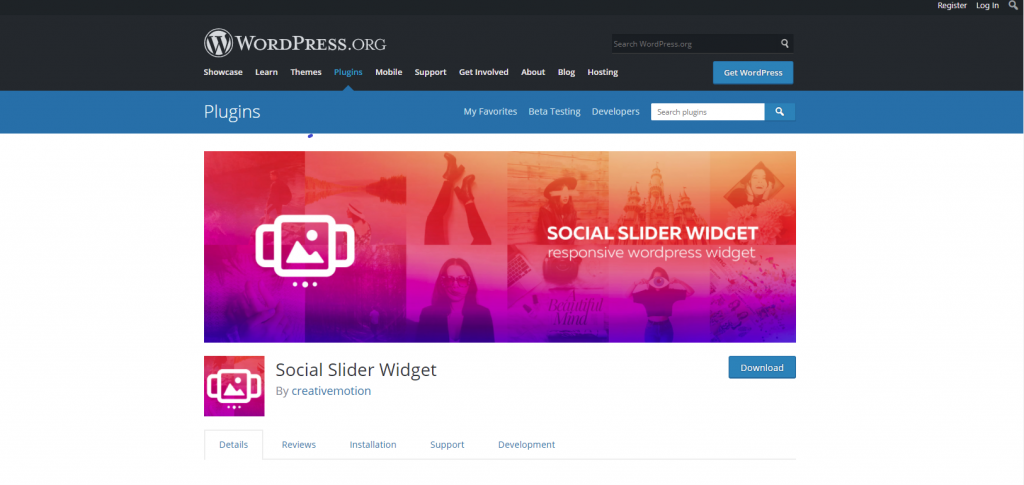This detailed screenshot from the WordPress.org website is showcased in a structured, black-themed box. The header of this box prominently features the WordPress logo—marked by a white circle containing a black "W". Below the logo, a navigation menu lists various sections: "Showcase," "Learn," "Themes," "Plugins," "Mobile Support," "Get Involved," "About," "Blog," and "Hosting." Adjacent to these options is a prominent blue button labeled "Get WordPress."

Beneath this black box lies a blue section focusing on plugins, offering categories such as "My Favorites," "Beta Testing," "Developers," and a search bar presented in white for easy navigation.

The background of the page is a collage composed of multiple images in varying shades of reds and purples. These images include two women, a close-up of a woman's legs, a person flexing their muscles, a girl standing with wind blowing through her hair and her glasses on, a mystical castle, and an abstract painting created by splashing paint directly from the brush.

Further down, the screenshot highlights a section dedicated to a plugin named "Social Slider Widget." Options for this plugin include "Download," "Details," "Reviews," "Installation," "Support," and "Development," providing users with comprehensive resources for their plugin management needs.